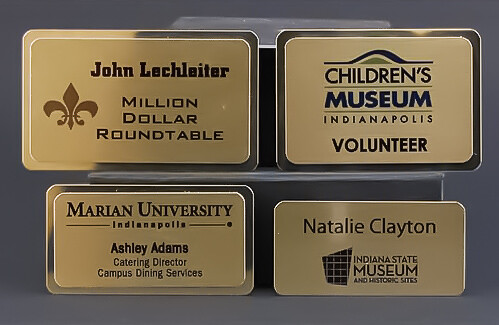This is a detailed photograph of four prestigious-looking gold name tags, possibly from an advertisement for custom employee pins. Each tag is meticulously designed and rectangular in shape. Starting from the upper left, the first name tag features a fleur-de-lis symbol, often associated with New Orleans and the Saints, and is inscribed with the name "John La Chocolater" and "Million Dollar Round Table." To its right, another tag has a black and green design at the top and reads "Children's Museum Indianapolis Volunteer." 

Below these, the name tag on the bottom left belongs to Marion University in Indianapolis and identifies "Ashley Adams" as the "Catering Director, Campus Dining Services." Finally, the name tag next to it indicates "Natalie Clayton, Indiana State Museum and Historic Sites." The name tags are uniformly displayed, though the background on which they are placed is difficult to discern.